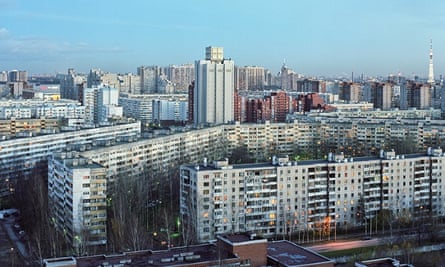The image is an elevated drone shot of a cityscape, capturing a large multi-story apartment complex prominently in the foreground. The complex, mostly white with many windows and balconies, forms an elongated triangular shape. It stretches from just above the bottom right corner to the center bottom, then angles upward diagonally, reaching a peak with the tallest building in the area. This tallest structure has a distinctive white facade with a small block at the top. To the left and back of the complex, more white buildings can be observed, with additional grey and red brick buildings to the right of the tallest one.

In the foreground, the apartment buildings encircle a central courtyard filled with tall trees, creating a secluded green space similar to how the Pentagon's structure encloses its interior. A road runs in front of the complex, adding to the urban setting. Beyond the complex, the background reveals a dense skyline of tall buildings under a blue sky with a few distant clouds and a low sun, casting a serene ambiance over the city.